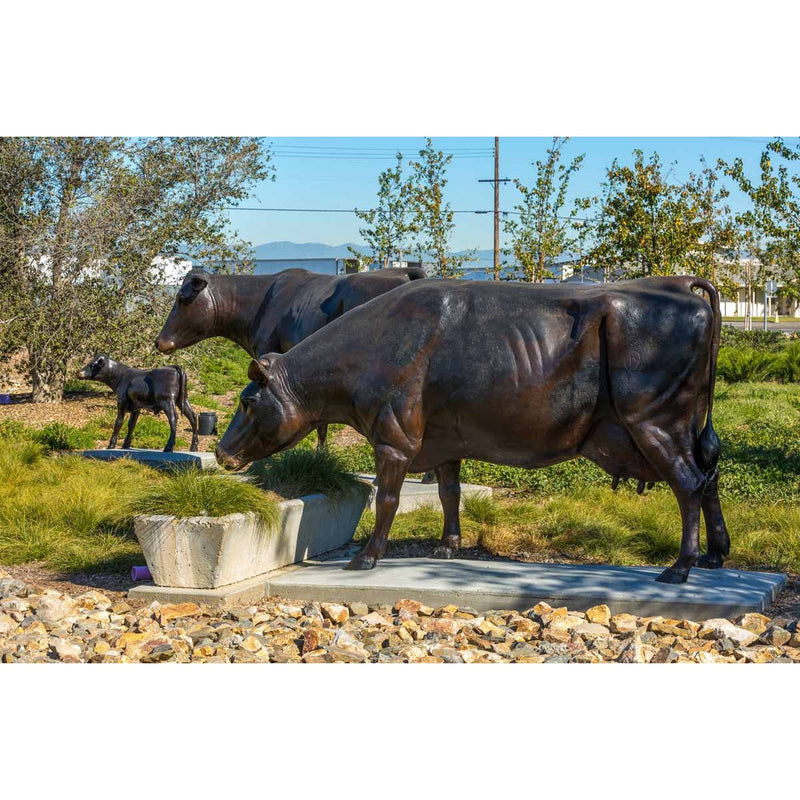This photograph captures a vivid scene of life-size, bronze statues of dairy cows installed in what appears to be a park or botanical garden. The focal point is a bronze cow in the foreground, positioned on a concrete base, seemingly feeding from a large concrete trough filled with real grasses, enhancing the lifelike appearance. Surrounding the trough is a landscape of rocky decorations. Behind the primary cow stands another large bronze cow accompanied by a calf, suggesting a family group. The backdrop features rows of trees, a hint of a road, and some houses, with distant mountains adding depth to the scene. The clear blue sky and rolling hills evoke a feeling reminiscent of California. The attention to detail in these statues makes them remarkable and lifelike representations of dairy cows, creating a serene and picturesque setting.